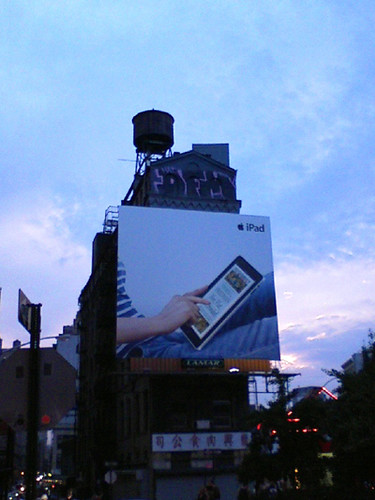The image depicts a large, square-shaped billboard mounted on the side of a brown building. The prominent feature of the billboard is a side view of a person reclining backward. Only the front of their body, part of their legs, and their forearms are visible. They're casually dressed in blue denim and a white and blue striped t-shirt, holding an iPad in one hand and interacting with it using their right hand. In the top right corner of the billboard, against a white background, the word "iPad" is clearly visible, accompanied by the Apple logo.

Below the billboard, the building displays a white banner with text written in a foreign, possibly Chinese, language. Additional structures around the billboard include the top part of a water tower. The street scene below is filled with activity, showcasing tail and headlights from vehicles, and a street sign on the left. The surrounding area is illuminated by lights, contributing to the impression that this location might be a bustling city potentially with a gaming or entertainment focus.

Above, the sky suggests either sunrise or sunset, with clouds and a horizon that is notably brighter, capturing the transitioning light of the day. The bottom right and left corners of the image reveal lit buildings, adding to the vibrant and dynamic atmosphere of the scene.